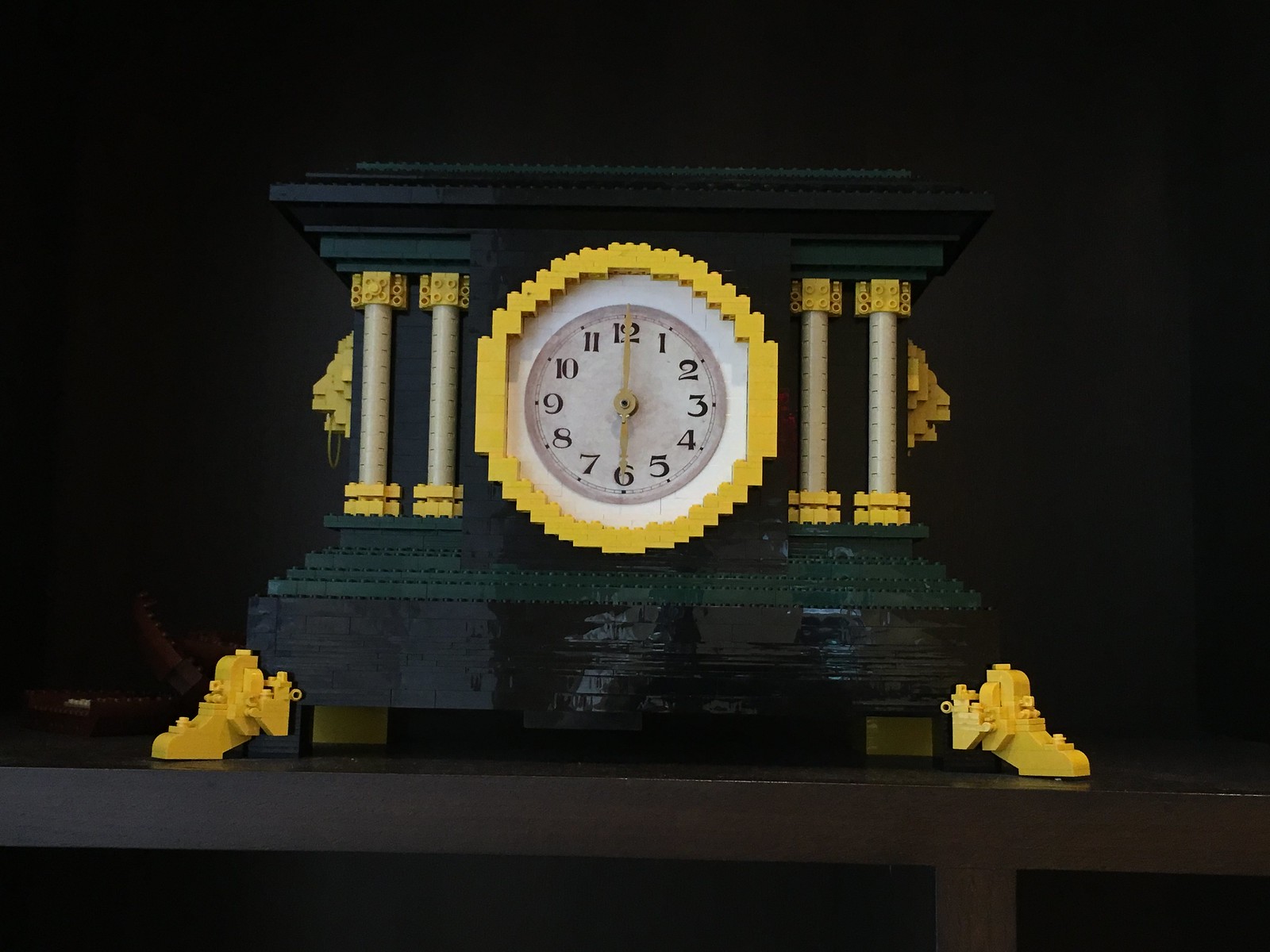The image depicts an intricate and detailed Lego clock that exudes the grandeur of a Greek palace. The clock is positioned atop a black shelf and showcases a visually striking, almost rectangular structure accentuated by layers of dark green Legos. The base features gold ornate feet at each corner, adding a touch of elegance.

The main clock housing resembles a stately Greek architectural design, complete with large, round columns on both sides of the clock face—two on each side. These columns are mainly gray, topped with yellow Lego braces. The housing itself also features additional layers of alternating dark green and yellow Legos, culminating in a top shelf that provides a rugged edge finish.

At the heart of this elaborate setup is the clock face, which is white with a yellow outline and gray rim. The numbers 1 through 12 are printed in clean, black font, while the time reads 6 o'clock, as indicated by yellow hour and minute hands. The clock face is surrounded by a gold frame that emphasizes its central position within the ornate structure.

The overall setup, which sits in dark shadow, adds to the dramatic and refined appearance of this Lego masterpiece.